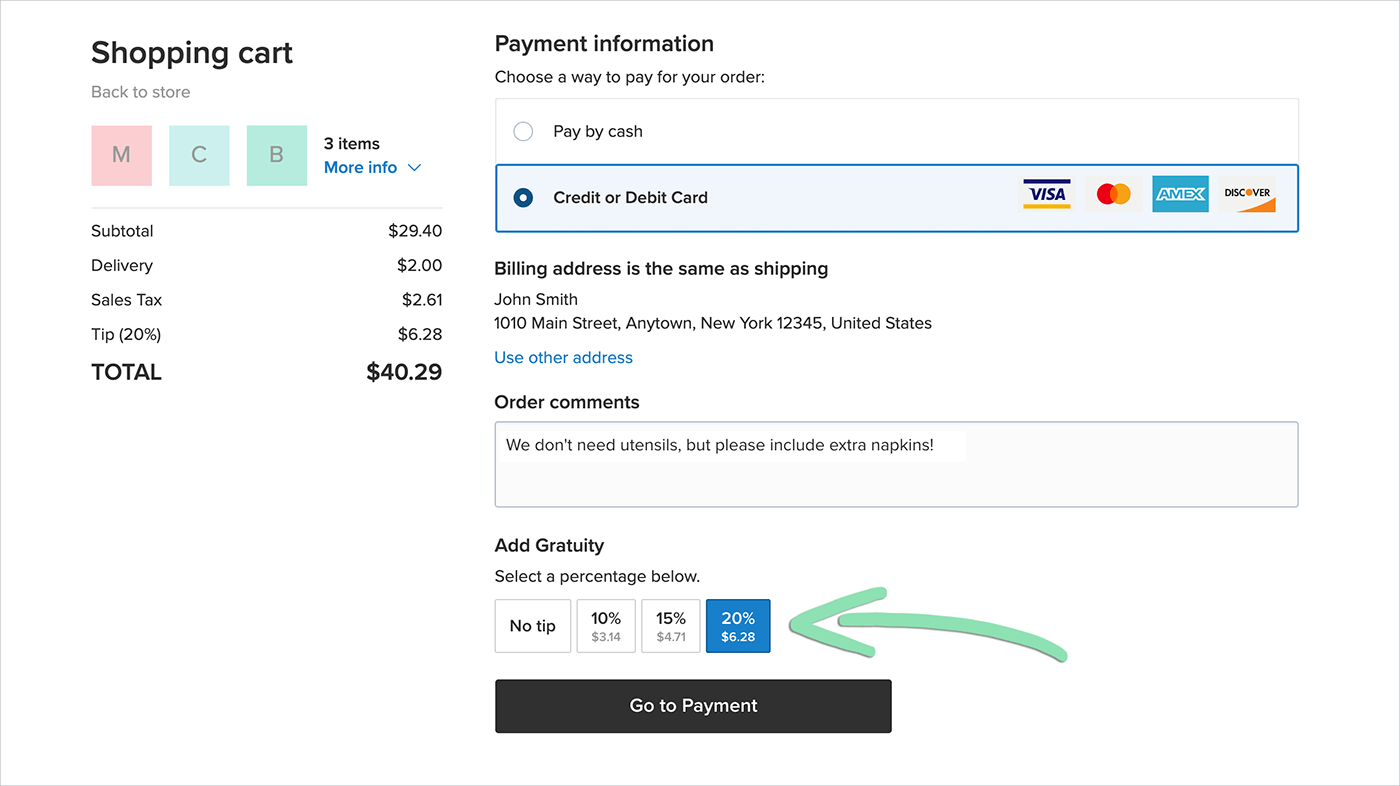The webpage features an online shopping cart interface for placing an order. At the top left, there is an icon of a shopping cart. Beneath it, a button labeled “Back to cart or store” is displayed. Adjacent to this, you can see the letters "M" in pink, "C" in green, and "B" in green. 

To the right, it indicates “3 items” with a link labeled “More info” in blue, which, when clicked, provides detailed information about each item. The cost breakdown is detailed with the subtotal being $29.40, a delivery charge of $2.00, sales tax amounting to $2.61, and a tip calculated at 20% which equals $6.28. The total amount stands at $40.29 and is prominently highlighted in bold compared to the other details.

Near the top, there is a section titled "Payment Information" asking users to choose a payment method for their order. Options include "Pay by Cash," with a checkmark option that turns into a blue dot when selected, or "Credit or Debit,” featuring logos of Visa, MasterCard, American Express, and Discover.

Beneath these options, there's a bold text stating "Billing address the same as shipping." Following that is an input area showing "John Smith" and the address "1010 Main Street, Inning Town, New York, 12345, United States." There is also a blue link below that reads "Use other address" for selecting an alternative address on file.

Further down, an "Order Comments" box includes the note “We don’t need utensils but please include extra napkins.” An "Add Gratuity" section allows selection of tip percentages: No Tip, 10%, 15%, or 20%, with each showing the corresponding amount. The 20% option is selected and highlighted in blue, with a hand-drawn green arrow pointing to it.

Finally, at the bottom, there is a black button labeled "Proceed to Payment."